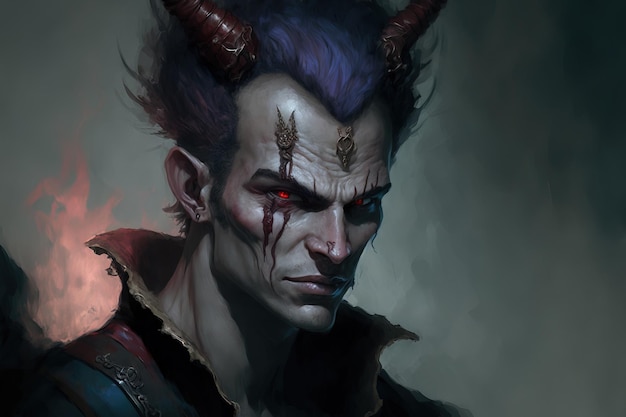The image depicts a detailed 3D rendered character with dark brownish skin, resembling a demon-like figure with human features. His most striking attributes are his glowing, bright red eyes and the two reddish-brown horns protruding from either side of his head. He has distinctive indigo-colored hair that is prominent and sharp in the middle, with bald patches on the sides, complemented by carvings and a red substance dripping down his cheeks. The character sports a maroon outfit with a striking red and gold turned-up collar. The background is predominantly gray and cloudy, with vibrant peach-colored flames on the left side, adding an intense, fantasy-like atmosphere to the scene.